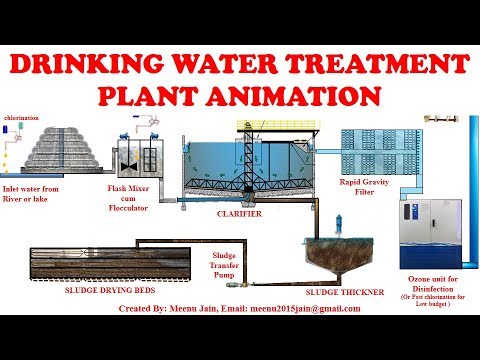The image is a detailed diagram depicting the stages of a drinking water treatment plant, titled "Drinking Water Treatment Plant Animation" in red text. The diagram, bordered by black bars at the top and bottom, illustrates the process from left to right. 

- On the far left, an inlet labeled "Inlet Water from River or Lake" shows water entering the system.
- The water first flows into a "Flash Mixer Cum Flocculator," a box equipped with multiple nozzles for mixing.
- From the mixer, water is directed into a large tank called the "Clarifier," which contains scaffolding and various internal equipment.
- The clarifier has two outputs: one leading to a "Sludge Thickener" and another to a "Rapid Gravity Filter."
- The rapid gravity filter is a brick-like structure that further purifies the water before it goes to an "Ozone Unit for Disinfection," a box-like tank ensuring the water is safe for consumption.
- Following disinfection, the treated water is ready for distribution as drinking water.

Separately, the sludge collected in the thickener is pumped via a "Sludge Transfer Pump" to "Sludge Drying Beds" for further processing and drying.

The text throughout is in red, and at the bottom of the diagram, the creator is credited: "Created by Manu Jane," with an email address provided as manu2015jane@gmail.com.